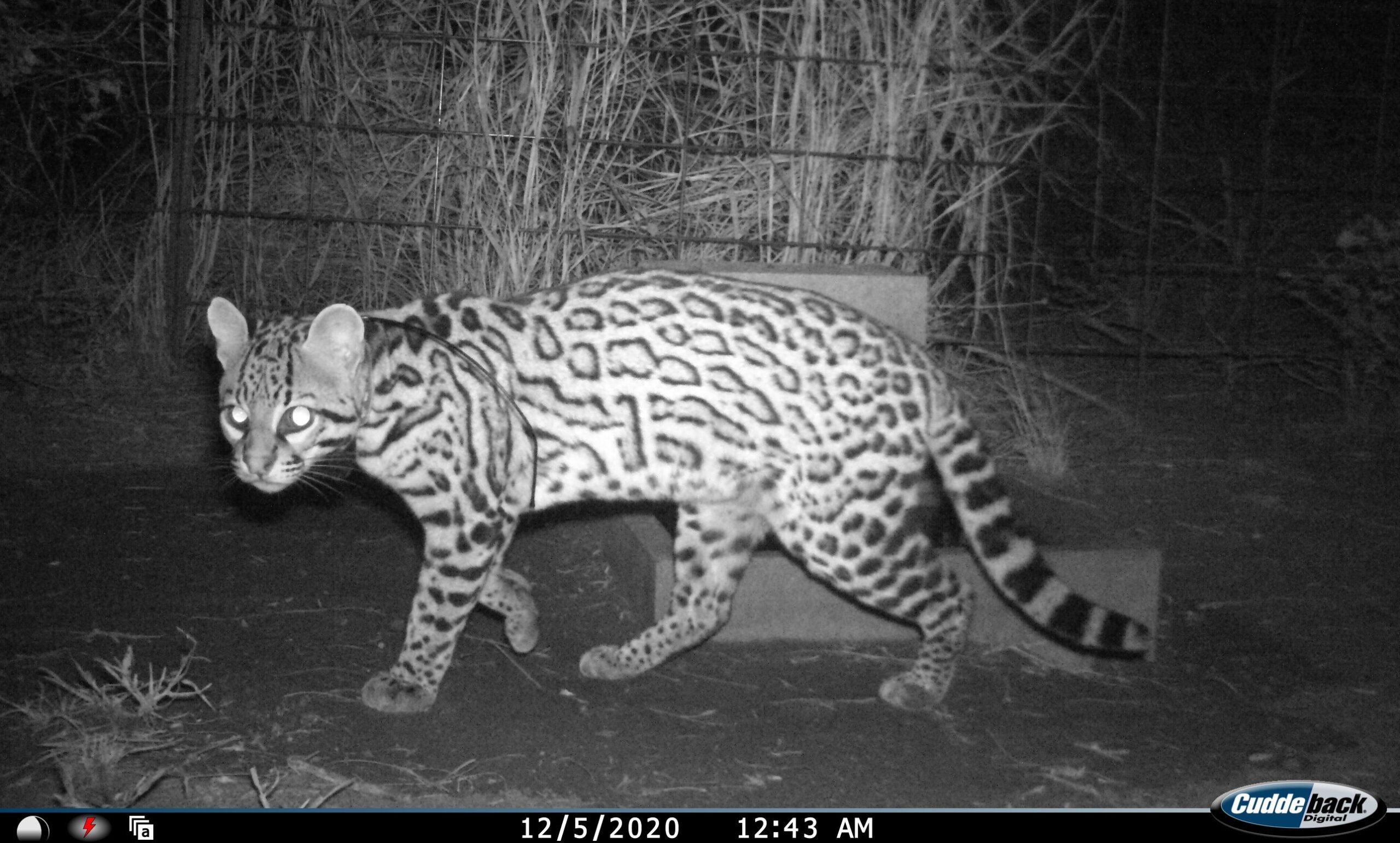This is a black-and-white nighttime photograph taken by a night vision camera, dated December 5th, 2020, at 12:43 AM. The picture features a medium-sized wild cat, possibly a leopard or cheetah, walking down a trail. The cat, with a distinctive striped tail, has its head facing to the left and possesses glowing eyes typical of nocturnal animals. The feline appears to be in motion against a backdrop of dried shrubs, wooden branches, and a fence, all set against a predominantly dark scene. At the bottom of the image, there is a black banner displaying the date and time, along with the label "CUDDE BACK original" on the bottom right.